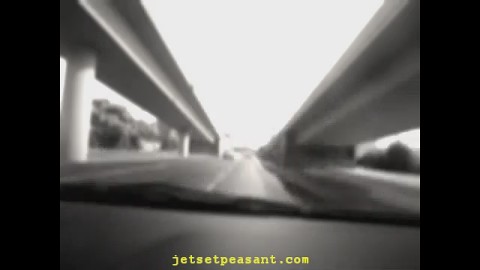A black and white photograph capturing a scene from a car's windshield, where part of the dashboard is visible. At the bottom center of the image, the text "jetsetpeasant.com" is displayed in a yellow lowercase font. The photo's borders on both the left and right sides are black, adding to its monochromatic aesthetic. The car is positioned underneath two gray cement stone bridges, each supported by sturdy beams. The image depicts a highway setting, with a white dotted line running along the center of the road. In the distance, other cars are seen traveling in the opposite direction. Beyond the bridges, a glimpse of lush green trees and shrubs adds a touch of nature to the composition.